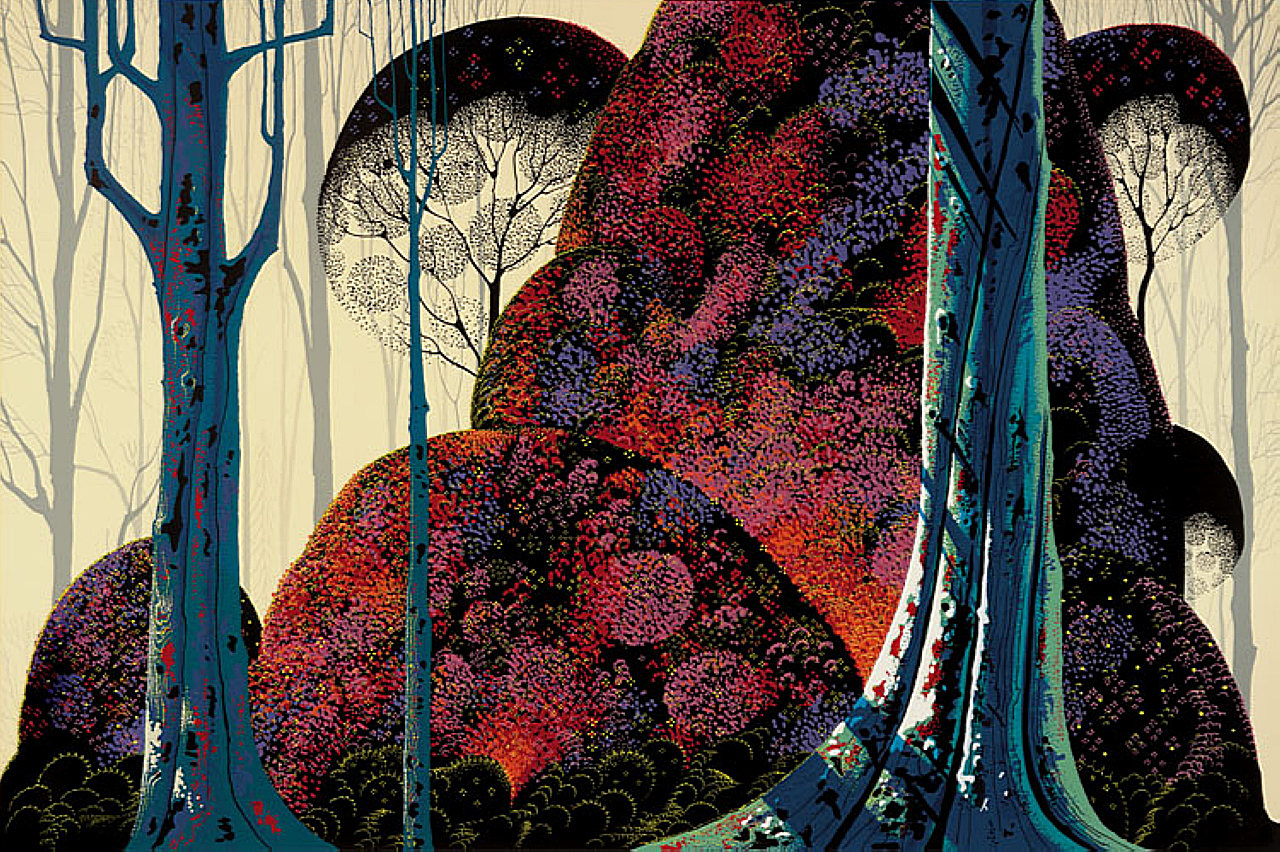This captivating piece of abstract digital art showcases a vibrant and surreal forest scene. Dominating the foreground are three tall, slender trees, primarily shaded in blue and green, adorned with splotches of red, white, and black. These trees stretch upwards, leafless, almost appearing twisted as they rise. Centrally located is an explosion of color, featuring a massive black bush teeming with tiny flowers in shades of red, pink, blue, purple, and yellow. The intricate flowers create a textured, almost spray-painted effect. The background sets a contrasting tone with a creamy yellow hue, accented by shadowy gray trees that loom distantly. Among these, some appear semi-transparent, their rounded tops densely blooming with similar multicolored flowers. This vivid, impressionistic landscape is highlighted by a soft haze, casting an ethereal light over the entire scene, enhancing the dreamlike quality of this unique artwork.